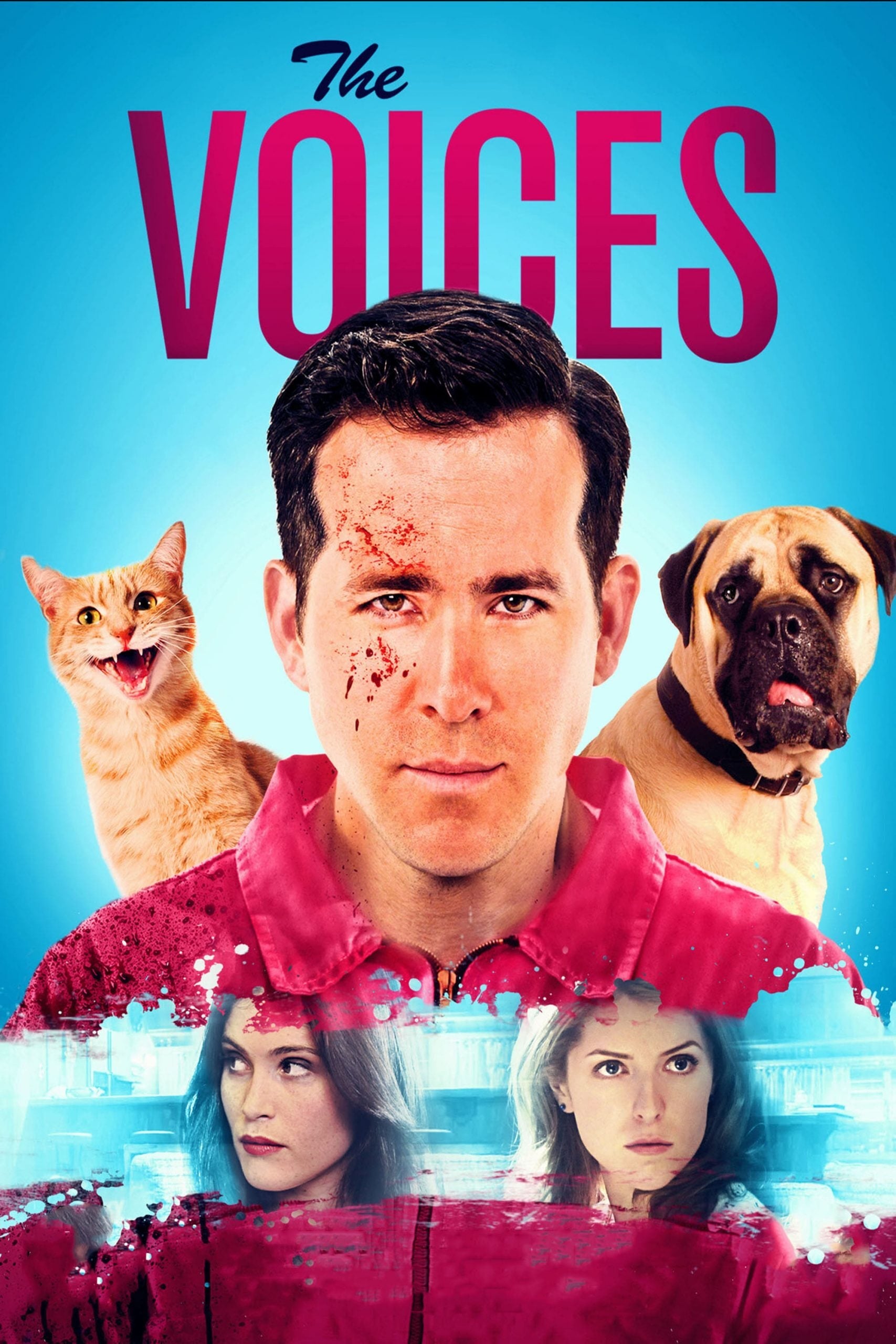This image is a movie poster or cover for a film titled "The Voices." The title features the word "The" in black stylized script, followed by "Voices" in bold purple uppercase letters. At the center of the poster is actor Ryan Reynolds, who is wearing a red collared shirt and has a smattering of blood on the left side of his face. To his left is an orange cat with its mouth open, and to his right is a light brown dog with black ears and a black snout. Superimposed across the chest area of his shirt are photographs of two women with long brown hair, both appearing intent and serious. The background is blue, making the central figures and text stand out vividly.